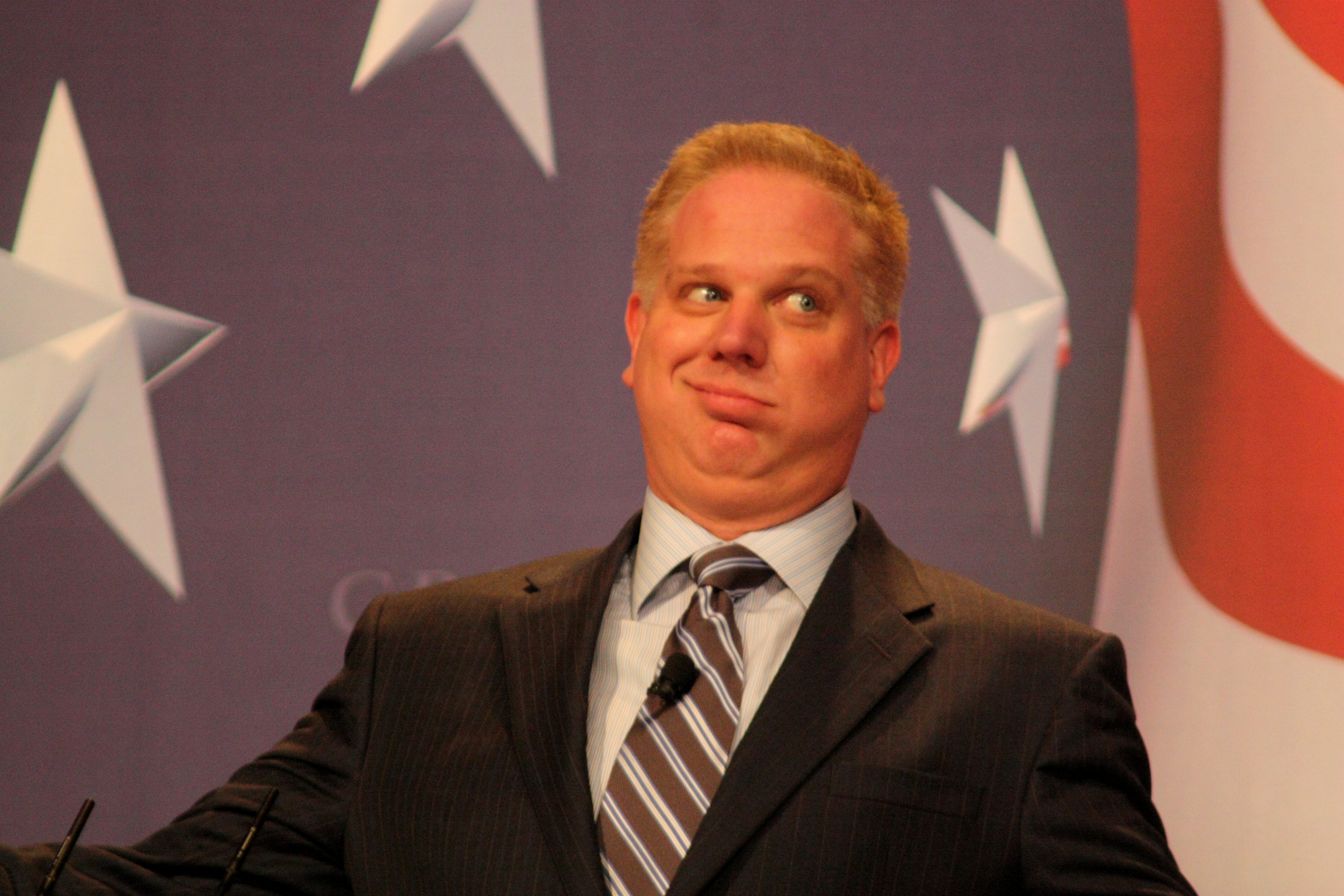This image is a close-up photograph of a middle-aged, apparently Caucasian man, likely at a debate or political event, set against a backdrop of the American flag with blue cloth, white stars, and a red stripe visible. The man has short blonde hair, light blue eyes, and is pulling a skeptical or amusing facial expression, slightly angling his mouth and looking off to the right. His expression causes his left cheek to puff out, giving him a somewhat unserious appearance. He is dressed in a black or dark gray pinstripe suit, a white dress shirt, and a tie with diagonal blue and white stripes. Additionally, there are two clip-on microphones visible—one blending into his suit near the bottom left and another attached to his tie. The background includes elements such as hanging white stars and a grayish hue, contributing to the ambiance of the event setting.